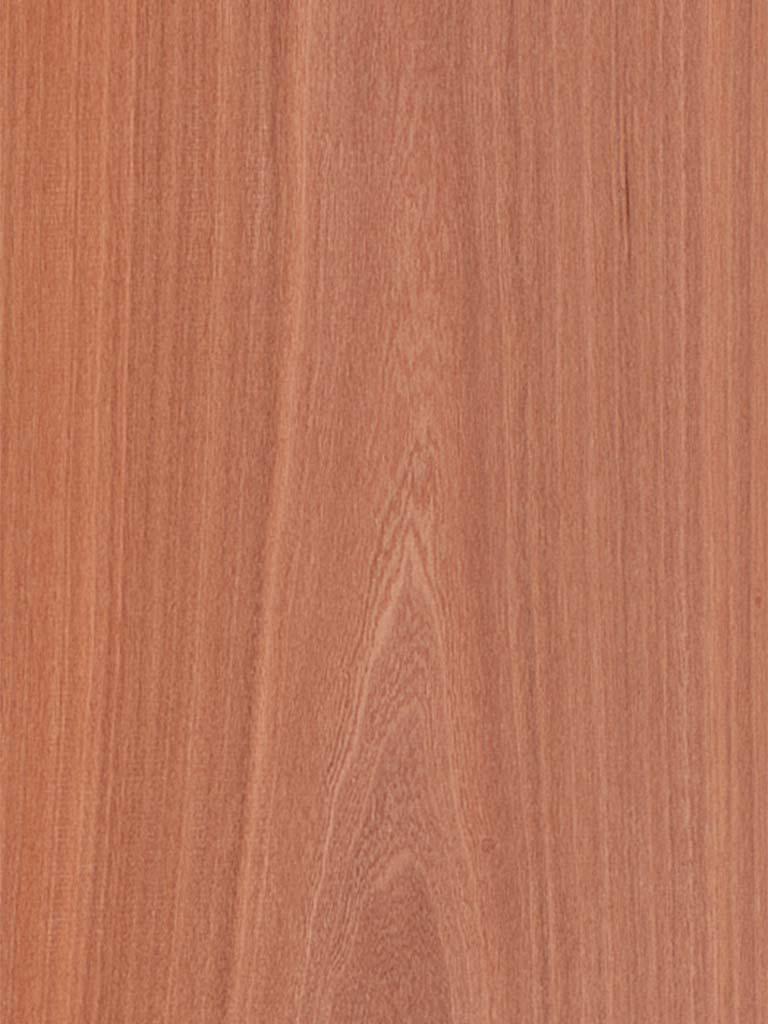This image is a detailed, close-up photograph of a finished piece of wood, likely from the top of a table or similar surface. The wood displays a rich brown color with variations of lighter and darker tones, and the grain runs vertically in straight, smooth lines. The surface appears to be well-sanded and finished, devoid of any imperfections, knots, or rough patches, although there’s a suggestion of an elongated triangular pattern possibly indicating a knot at the center. The overall appearance is highly polished and has a deep, honey-like hue, giving the impression of an artificial or manufactured woodgrain, similar to that found on desktops or peel-and-stick contact paper. The focus of the image is entirely on the wood's texture and grain, with no other objects, text, or numbers present.